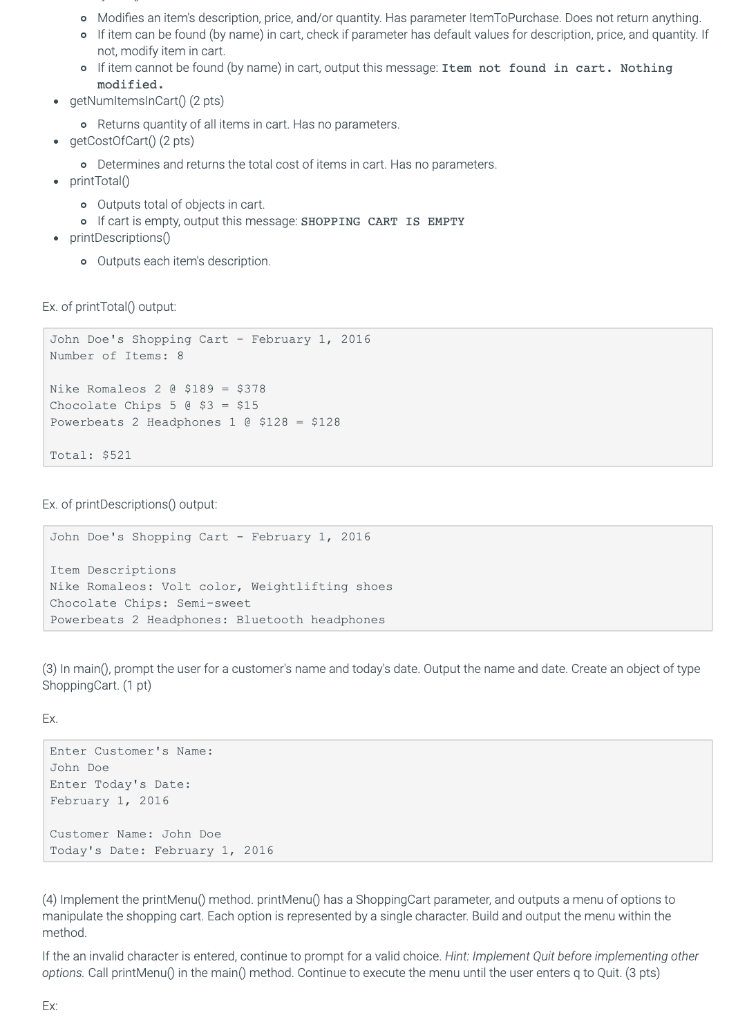This image showcases a detailed printout related to an item management system, likely a part of software or a documentation manual. At the top, the document begins with a bulleted list explaining various functions and their behavior:

- **Modify Item Description/Price/Quantity:** 
   - **Bullet:** Modifies an item's description, price, or quantity based on provided parameters. Does not return any value.
   - **Bullet:** If the item can be located by name in the CART, the system checks for default values for description, price, and quantity parameters.
   - **Bullet:** If the item is not found by name in the CART, it outputs the message, "Item not found in CART. Nothing modified."

The document proceeds with multiple additional entries, explaining different functionalities:
- **GetNumItemsInCart:** Returns the total quantity of all items in the CART. This function has no parameters.
- **DetermineTotalCost:** Calculates and returns the total cost of all items in the CART. This function also has no parameters.
- **OutputEachItemDescription:** This function outputs the description of each item.

Towards the bottom, the document has a gray-shaded section showcasing an example of a "Print Total Output." This example includes specifics such as:

- **Header:** John Doe's Shopping Cart, February 1, 2016
- **Details:** 
  - Number of items: 8
  - Item details with quantities and prices:
    - Nike Romaleos: 2 at $189 each, totaling $378
    - Chocolate Chips: 5 at $3 each, totaling $15
    - Powerbeats 2 Headphones: 1 at $128, totaling $128
  - **Total Cost:** $521

The document repeats this information for another order under John Doe, implying it showcases different order entries, complete with item details, quantities, and total costs. This structured layout helps in visualizing how to process and verify customer orders through the system, with clear prompts for different customer names and order details.